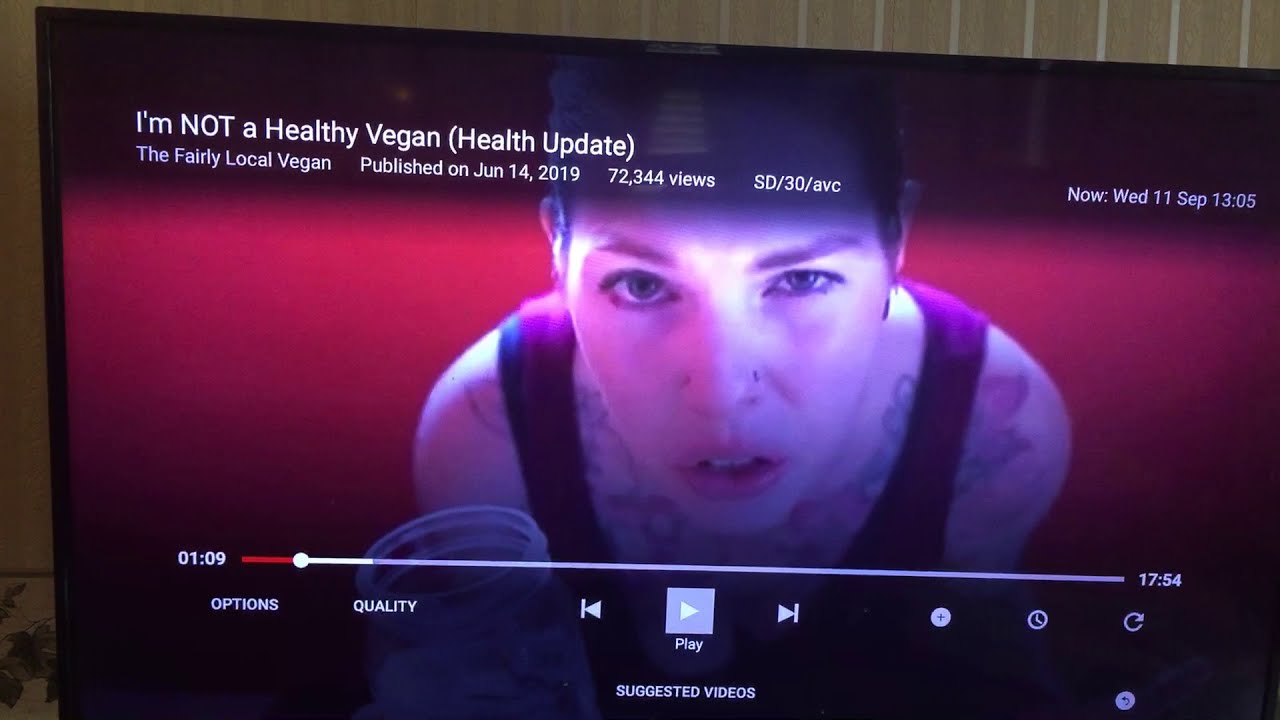The photograph captures a paused video on a LED TV screen, situated within a room featuring a brown wall with vertical lines. The TV's sleek black frame is visible, and portions of the room are glimpsed around it. On the screen, a YouTube video titled "I'm Not a Healthy Vegan: Health Update" from the channel Fairly Local Vegan, published on June 14th, 2019, is displayed. The paused video shows a woman with short hair and faint tattoos, wearing a maroon tank top, looking intently at the camera with one eyebrow raised. She is holding a clear jar in her hand against a bright magenta background. The video is paused at the one minute and nine second mark, with video control buttons, including a play button and a red progress bar, visible at the bottom of the screen.